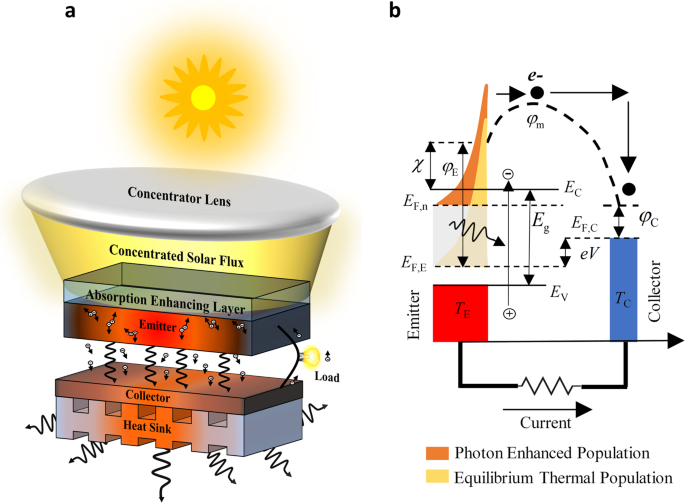This image features a detailed scientific diagram related to solar power, presented on a white background. The diagram is divided into two sections labeled 'A' and 'B'.

In section 'A,' the diagram illustrates the process of solar energy concentration and conversion. At the top left corner, there is an image of a sun emitting a beam of yellow light. This light is focused through a white oval labeled "concentrator lens," which then directs the "concentrated solar flux" onto a series of components below:

1. A transparent rectangular layer labeled "absorption enhancing layer."
2. A darker, heat-emitting layer labeled "emitter," depicted with a color gradient from red in the center to orange at the edges. This layer features moving dots with arrows, indicating the flow of energy.
3. An empty space labeled "load," where squiggly lines and dots representing the energy transition are observed, along with a lit light bulb, suggesting the conversion of solar energy into usable electricity.
4. A solid layer beneath the load labeled "collector."
5. A lattice-shaped, gray object labeled "heat sink," which emits squiggly lines symbolizing the dissipation of heat.

In section 'B,' the diagram delves into the theoretical framework behind the energy conversion process. This part includes:

1. An array of black arrows, dotted arches, and mathematical equations.
2. Charts and graphs illustrating the relationship between components such as the "emitter" and "collector."
3. Labels indicating "current," flowing to the right, and a key explaining the different populations: "photon enhanced population" (brown) and "equilibrium thermal population" (yellow).

These detailed visual and theoretical representations provide a comprehensive understanding of how solar energy is concentrated and converted into electricity.